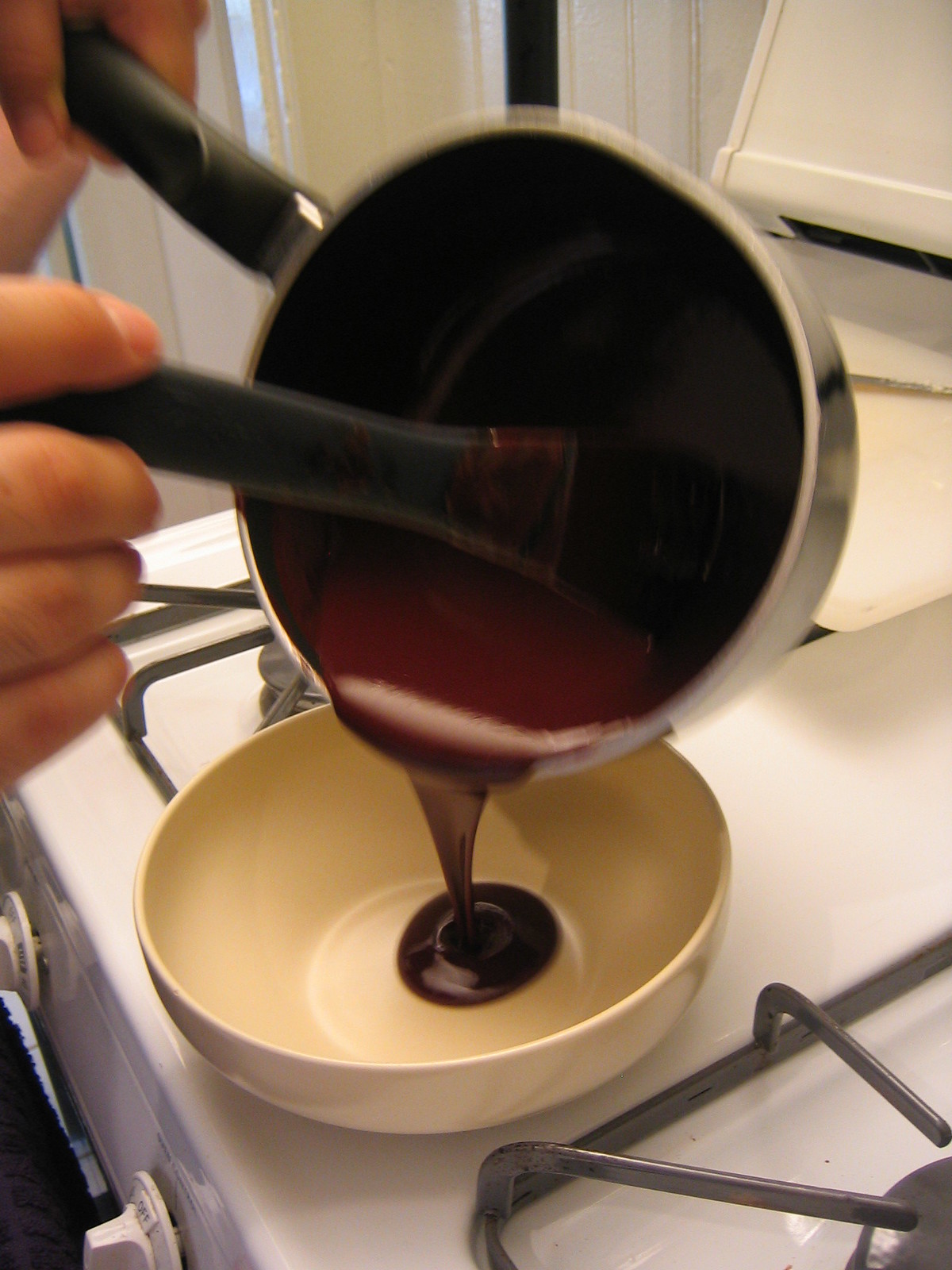In this detailed indoor photograph, the scene captures the moment someone is pouring what appears to be melted chocolate sauce from a small black saucepan into a white or beige bowl. The photo is taken from an overhead angle, allowing a comprehensive view of the white gas stovetop, which features metal trivets and burners. 

One hand, visible at the top right corner, tilts the saucepan to facilitate the flow of the thick, creamy brown chocolate into the bowl positioned centrally on the stove. Meanwhile, the other hand, visible with four fingers, uses a dark gray pastry brush or spatula to scrape the remaining chocolate from the saucepan, ensuring all of it makes its way into the bowl.

The backdrop includes white walls and an indiscernible black object. The stovetop's silver turn knobs and metal circle burners add a vintage touch, highlighting the old-school design of the cooking setup. The overall composition provides a tactile sense of the cooking process, focusing on the rich texture of the melted chocolate as it pours into the bowl.